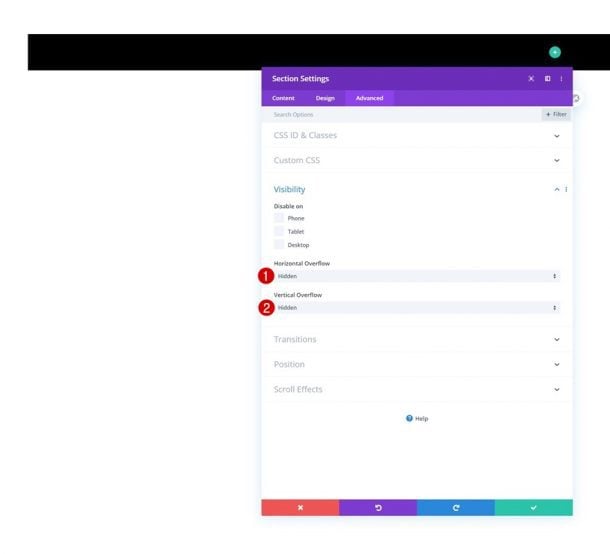Screenshot of a section settings menu with various configuration options. The menu is divided into multiple tabs: Content, Design, and Advanced. Within the Advanced tab, settings include fields for CSS ID and classes. Dropdown menus are available for custom CSS and visibility settings. Visibility options include disable on phone, tablet, or desktop, each indicated with corresponding checkboxes. Additional settings are present for horizontal overflow marked as "one" or "hidden," and vertical overflow set to "hidden." There are options for transitions and scroll effects, marked with a question mark and a blue circle for help. Action buttons include a red X for delete, a refresh icon inside a purple square, another refresh icon inside a blue square, and a check mark inside a green square for confirmation.